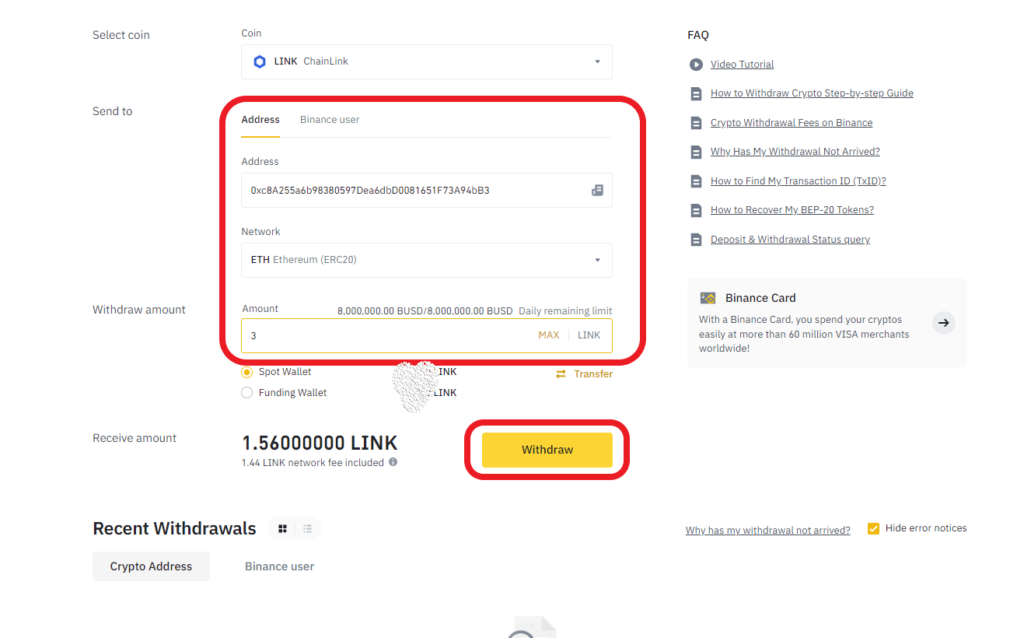The image depicts a withdrawal page from a cryptocurrency website. At the top, there is an option to select the type of coin for the transaction, with "Chainlink (LINK)" chosen in this instance. A small, blue hexagonal logo representing Chainlink is next to the coin name. The user appears to be transferring funds to someone else, as indicated by the "Send to" field where a wallet address is entered. The transaction is set to occur on the Ethereum network.

The user is sending 3 LINK, specified in a yellow-highlighted "Amount" field that includes a "MAX" button. Next to this field is the term "LINK," reiterating the cryptocurrency in use. Below, the "Spot Wallet" option is selected, marked with a bubble-shaped icon resembling a heart made of soap suds, likely an addition by the person who shared the screenshot.

The "Amount to be received" field indicates that the recipient will get 1.56 LINK, after fees or deductions. The withdrawal can be confirmed by clicking a yellow rectangle labeled "Withdraw" in black font. Key fields, such as "Send to" and "Withdraw Amount," are highlighted with red rounded rectangles, emphasizing their importance.

The bottom part of the page shows details of recent withdrawals, including information like the crypto addresses used and the Binance user associated with those transactions.